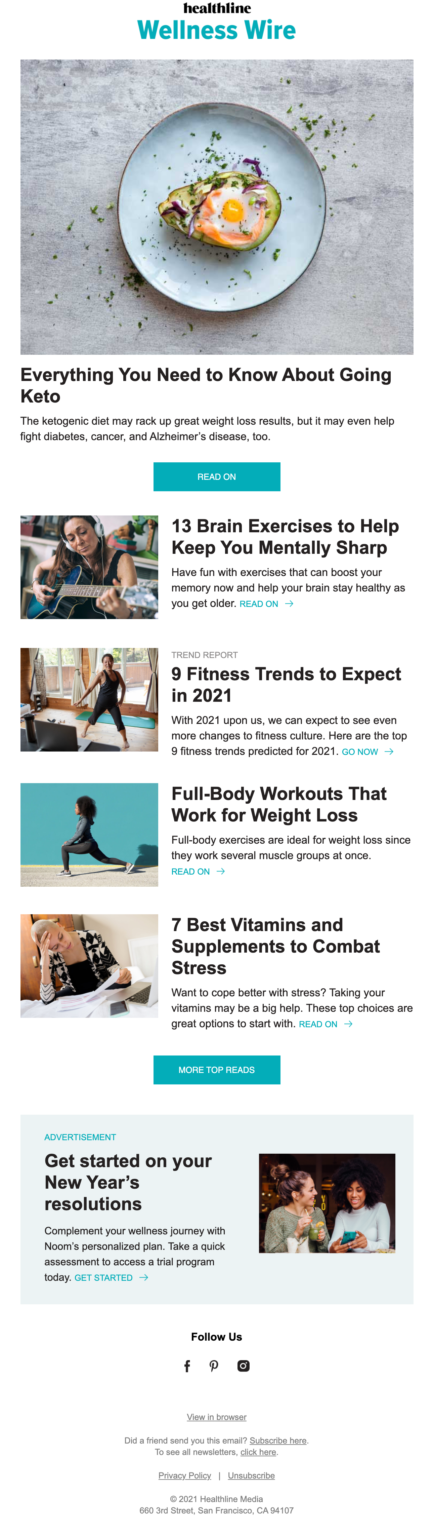The webpage being described in the image appears to be a health and wellness site named "Wellness Wire." At the top, the title "Headline Wellness Wire" is displayed prominently, with "Headline" in black text and "Wellness Wire" in a light blue or light green hue. Below the title, there is an image featuring a white plate containing a keto-friendly meal that includes eggs, avocado, and some green vegetables. Underneath the image, a bold headline reads: "Everything You Need to Know About Going Keto." 

The article summary explains that the ketogenic diet not only promotes significant weight loss but may also aid in combating diabetes, cancer, and Alzheimer's disease. A blue "Read On" button invites viewers to explore the article further.

Further down the page, another headline reads: "Getting Brain Exercises to Help Keep You Mentally Sharp." The brief description encourages readers to engage in fun exercises that can enhance memory and maintain brain health as they age. A "Read On" prompt directs users to more information.

Another subsection highlights "9 Fitness Trends We Expect in 2021," predicting significant changes in fitness culture for the upcoming year. Readers are encouraged to discover the top fitness trends via a "Go Now" button.

Following this, an article titled "Full Body Workouts That Work for Weight Loss" discusses the benefits of full body exercises which target multiple muscle groups simultaneously, making them effective for weight loss.

The next headline, "7 Best Vitamins and Supplements to Combat Stress," offers advice on vitamins that can help manage stress, recommending some top choices to start with.

At the bottom of the page, additional links are marked under "More Top Rated." There is also an advertisement section encouraging readers to "Get Started on Your New Year's Resolutions" with a focus on health, care, and wellness.

Overall, the webpage appears to be a comprehensive resource for various aspects of health and fitness, providing readers with valuable information, tips, and trends to help them lead healthier lives.